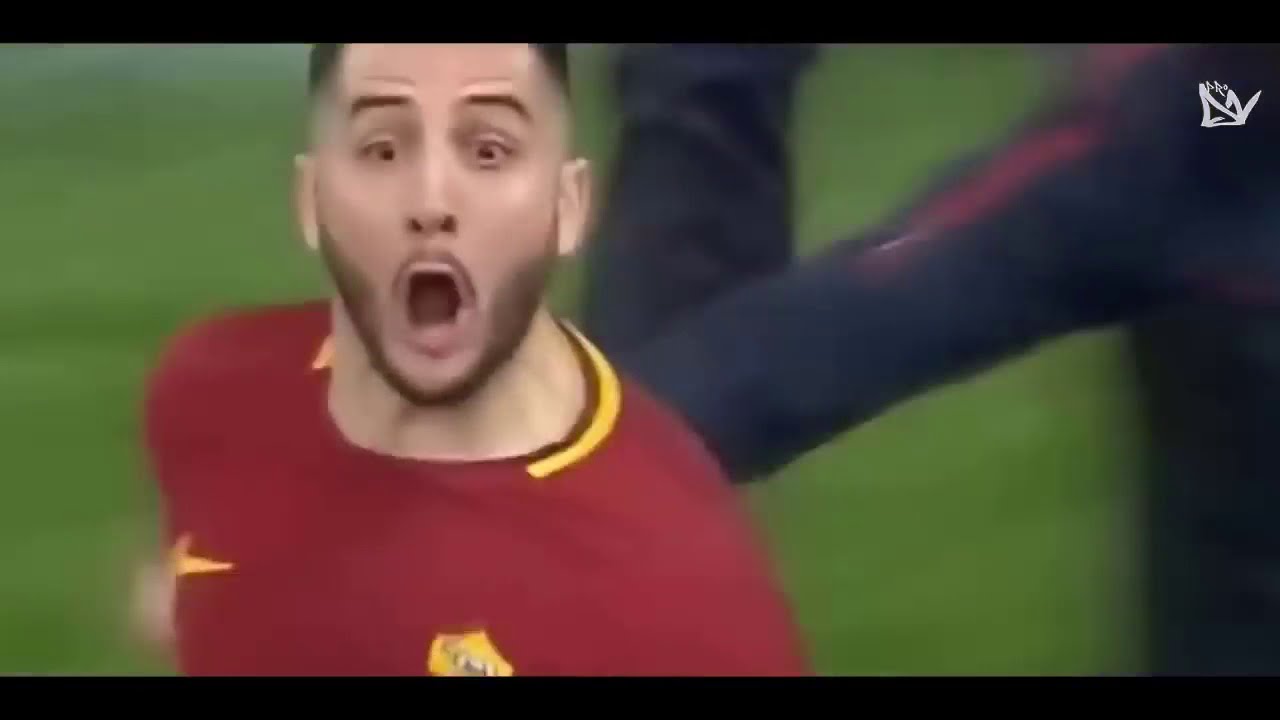The image captures a dynamic moment during a sports game, likely soccer or football, set on a green outdoor field. The focal point is a man with short black hair and dark facial hair, sporting a nicely cut fade. He is wearing a light maroon jersey with yellow accents, including a Nike logo and a symbol on the left breast. His mouth is wide open in an oval shape, and his eyes are wide with raised eyebrows, conveying intense surprise or excitement, possibly due to a victorious moment. The photo shows him from his forehead down to his chest. 

In the background, there appears to be another player, partly visible with black pants featuring a maroon stripe and what seems like the right side of their body in a black jacket. The image has black strips at the top and bottom, and a blurry logo in the upper right corner that resembles a white crown with arrows pointing upward. Despite the blur, the setting, expressions, and attire detail a moment of high energy and emotion on the field.